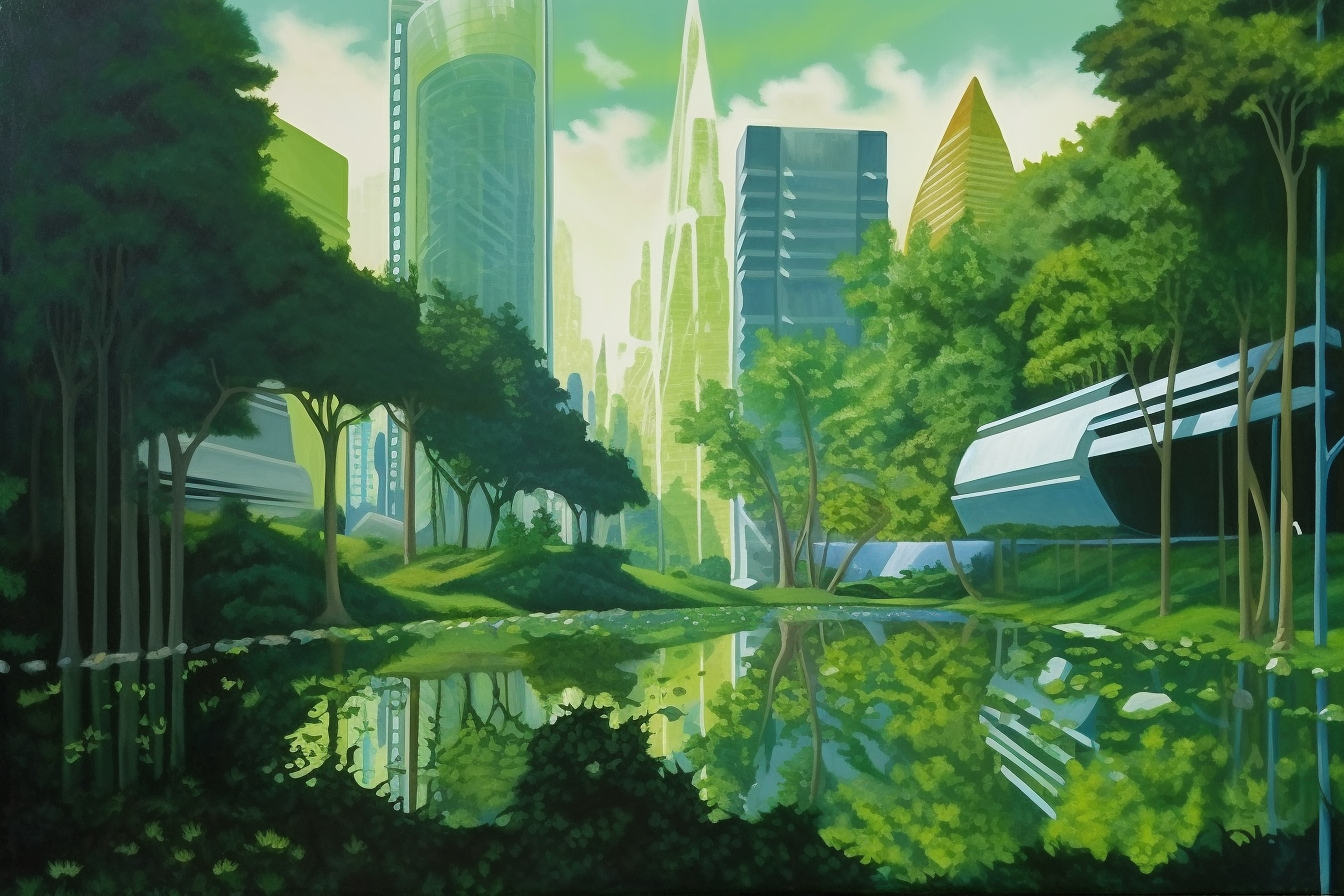This image is a highly detailed, artistic rendering of a futuristic cityscape featuring a centrally positioned lake or pond. The water in the foreground mirrors the surrounding elements, reflecting trees, shrubs, and the skyline in its calm surface. Flanking the lake on both sides are thin, glimmering trees with green leaves, and dark bushes that add depth to the scene. The background reveals towering, glass-like skyscrapers, which are silver and translucent, giving a modern, ethereal quality to the city. Some buildings exhibit green accents, creating harmony with the sky, which has a blend of blue and green hues filled with white clouds.

Prominently positioned in the middle of the image is a unique futuristic structure with a white, curved roof, resembling a tubular building. Another significant building stands nearby, shaped like a white, clear crystal or shard of glass, sharp at the top. A plain gray, silver rectangular skyscraper is visible next to it, adding contrast to the scene. Further in the background, a pointed, tan-colored building resembling a pyramid rises against the skyline. The overall scenery depicts a serene park nestled within a cutting-edge, modern city, enhanced by subtle tones of green and tan throughout the composition.